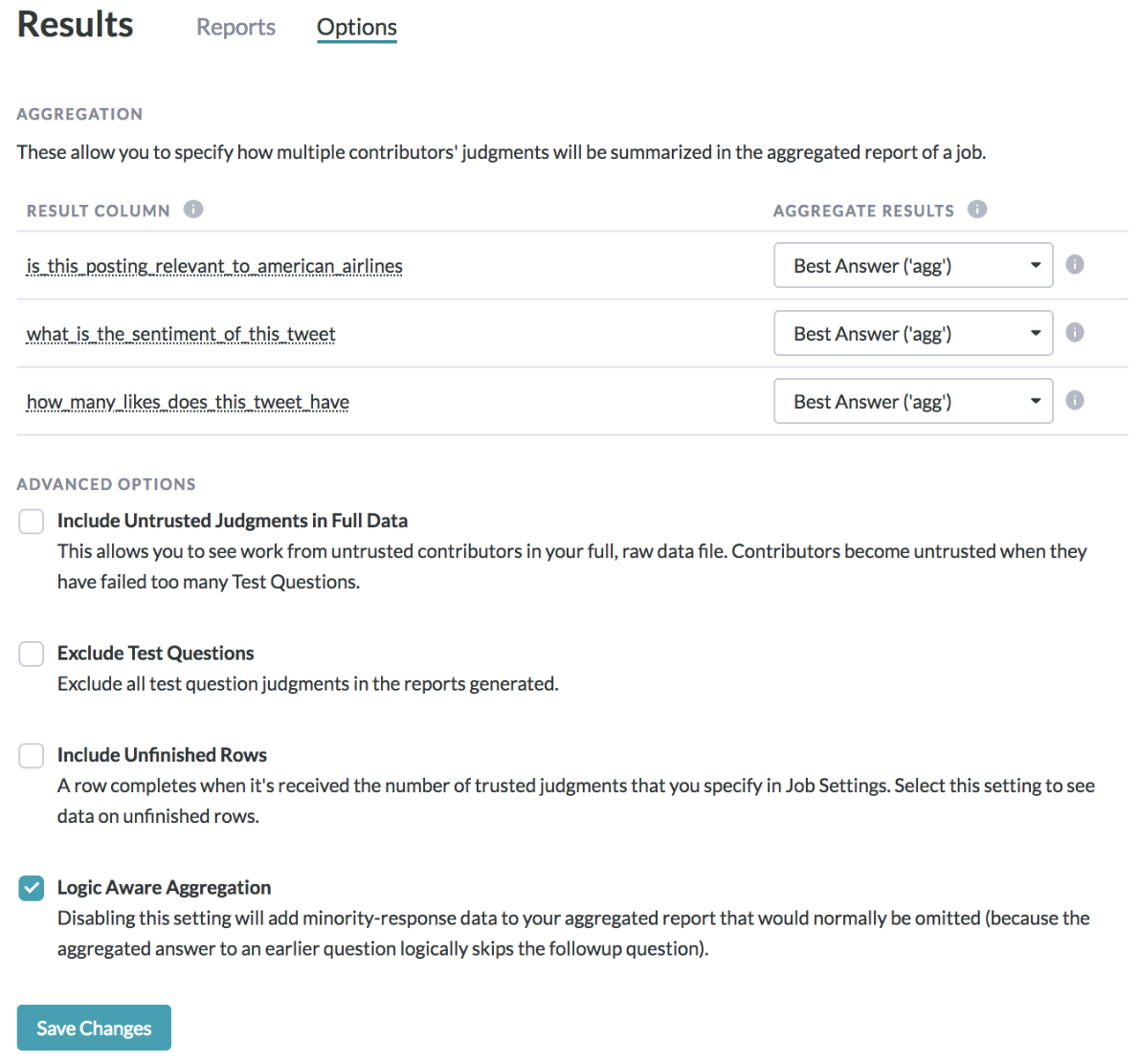The screenshot depicts a section of a website interface with a clean, white background. Positioned at the top in bold and larger font is the word "Results," with a capital 'R'. To the right, there are two options: "Reports" and "Options." The word "Options" is underlined in blue, marked with a capital 'O', and appears in a bold print.

Directly below "Results," there is the heading "AGGREGATION," displayed in all capital letters. This section explains that it allows users to specify how multiple contributors' judgments will be summarized in the aggregated report of a job. Further down, the term "Result Column" is mentioned, followed by "Aggregate Results," which has a small banner containing a drop-down menu.

Continuing downward, there is a section titled "Advanced Options" accompanied by several selectable items. Each option has a small square checkbox in front of it. The options listed include:
1. Include Untrusted Judgments in Full Data
2. Exclude Test Questions
3. Include Unfinished Rows
4. Logic Aware Aggregation

The "Logic Aware Aggregation" option is selected, as indicated by its teal color and a white check mark inside the checkbox.

Beneath these options, there is a teal-colored rectangle button with the text "Save Changes" written in white.